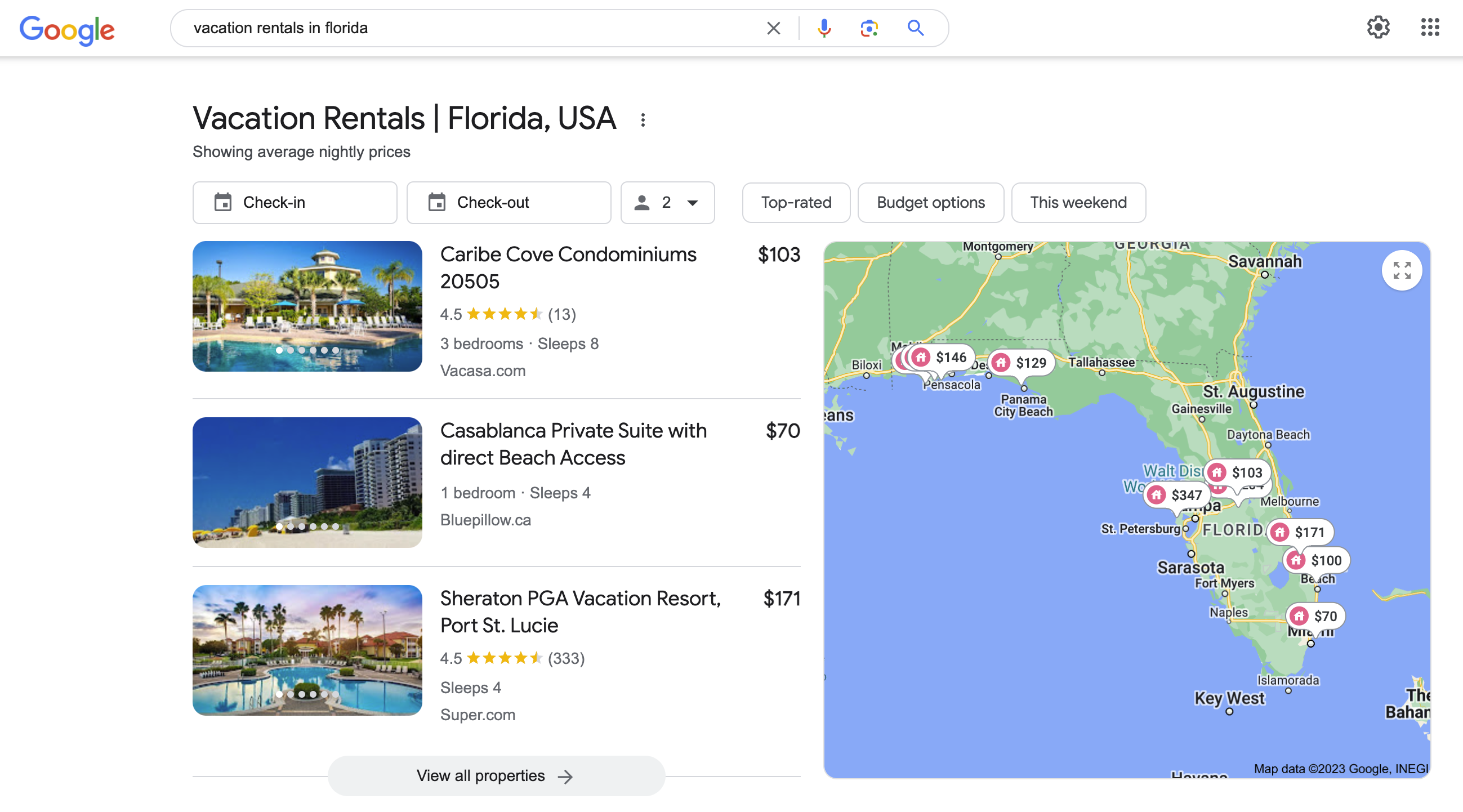The image depicts a Google search results page for "vacation rentals in Florida." At the top left corner, the Google logo is prominently displayed. The search query "vacation rentals in Florida" is typed into the search bar, with a suggestion beneath it reading "vacation rentals in Florida, USA." Below, a notice states that the results are showing average nightly prices. 

Six filter boxes are aligned horizontally, labeled from left to right: "Check-in," "Check-out," "Number of people," "Top rated," "Budget options," and "This weekend." 

On the left side of the page, three top-rated vacation properties are listed:
1. Caribbee Cove Condominiums, with a nightly rate of $103. A photo of a pool area represents this property.
2. Casablanca Private Suite with direct beach access, priced at $70 per night, illustrated with an image of a beachfront view.
3. Sheraton PGA Vacation Resort Port St. Lucie, costing $171 per night, shown with a photo featuring a pool area surrounded by palm trees.

Below these listings, there is an option to "View all properties."

On the right side, a detailed map of Florida showcases the blue ocean adjacent to the landmass, with markers indicating the locations of various vacation rentals throughout the state. 

This comprehensive layout provides a clear overview for users searching for vacation accommodations in Florida.